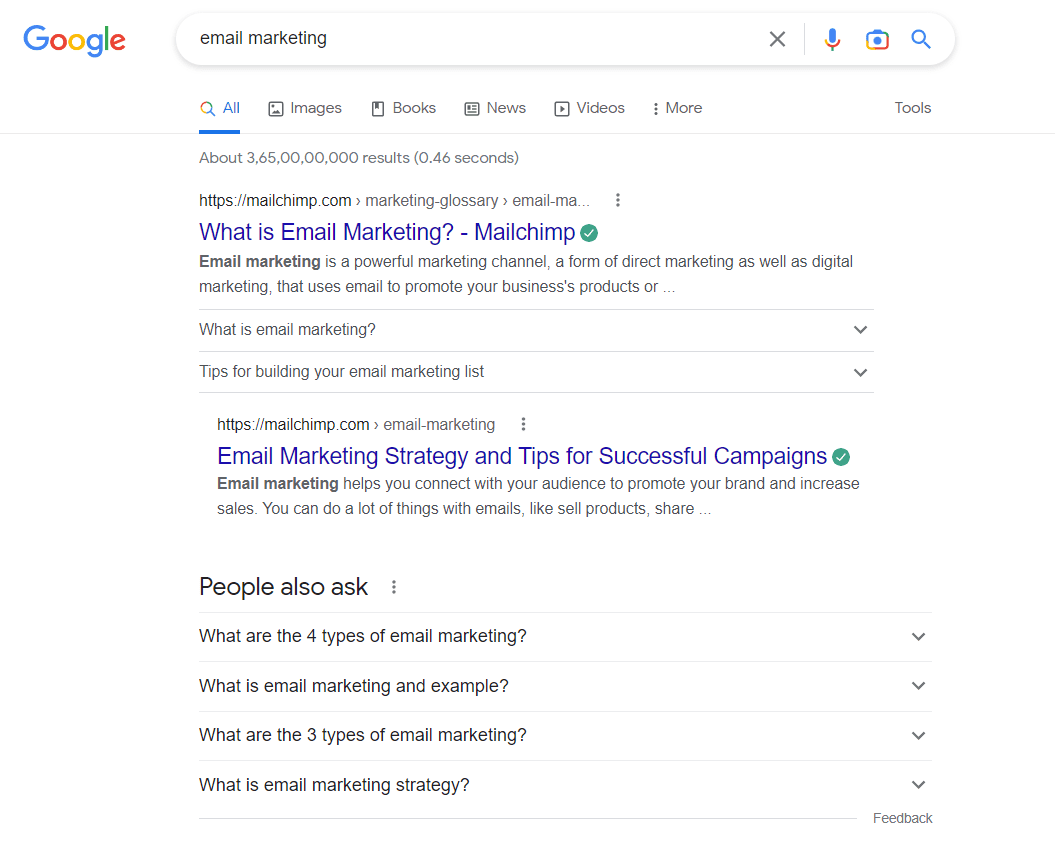This image captures a Google search results page for the term "email marketing." The backdrop is a clean, white interface featuring the iconic Google logo with its standard colors: blue, red, yellow, and green. The search results are notably sparse, with only two entries. Both entries prominently feature MailChimp, a well-known email marketing service, marked with green checkmarks indicating trustworthiness. 

Adjacent to the search results, there's a "People also ask" section listing common queries such as "What are the four types of email marketing?" and "What is an email marketing strategy?" Intriguingly, there are no ads displayed on this page, which is unusual for such a high-demand keyword. The page suggests an overwhelming volume of information is available on the topic, quantified in billions or trillions of results. Despite the lack of ads, the clean and simple design focuses attention clearly on the organic search results and related questions.